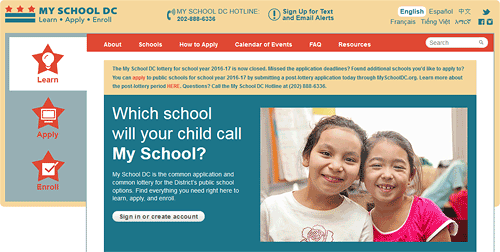This image is a screenshot from the MySchoolDC website. At the upper left-hand corner, the name "MySchoolDC" is prominently displayed in all capital letters with a greenish-blue font. Beneath the title, in thinner font, are the words "Learn. Apply. Enroll." separated by dots. To the left of the title, there are two horizontal lines stacked above each other, with three red stars positioned above the lines.

In the same upper bar, there is a phone number for the school, an option to sign up for text and email alerts, and language selection options for English, Spanish, and French. Social media icons for Twitter and Facebook are also visible on this bar.

On the left side of the website, a vertical menu displays the tabs labeled "Learn," "Apply," and "Enroll." The main portion of the webpage, located on the right side, features the text "Which school will your child call My School?" accompanied by a picture of two children standing side by side, looking directly at the camera.